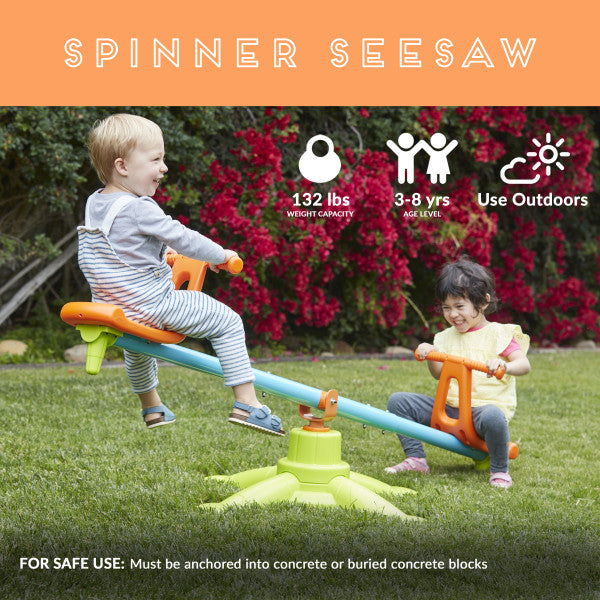In this advertisement image, we see a playful scene featuring two children on a brightly colored seesaw, set in an outdoor yard of lush green grass. The seesaw has a blue frame with two orange seats. On the left side, a blonde-haired boy dressed in a gray outfit and sandals is lifted into the air, while on the right, a girl with dark black hair and dressed in a pink shirt layered with a yellow shirt and gray pants, balances opposite him. Both children are laughing and having a good time. Overhead, in a peach-colored strip with a distinctive white font, it reads "Spinner Seesaw." Additional text at the top-right corner indicates a 132 pounds weight capacity, age suitability of 3 to 8 years, and a reminder to use outdoors. For safe use, it specifies that the seesaw must be anchored into concrete or buried concrete blocks. In the background, vibrant red flowers, possibly roses, grow on the vines, adding to the cheerful and lively atmosphere. The image communicates the product specifications clearly with relevant icons, making it suitable for packaging or advertisement purposes.